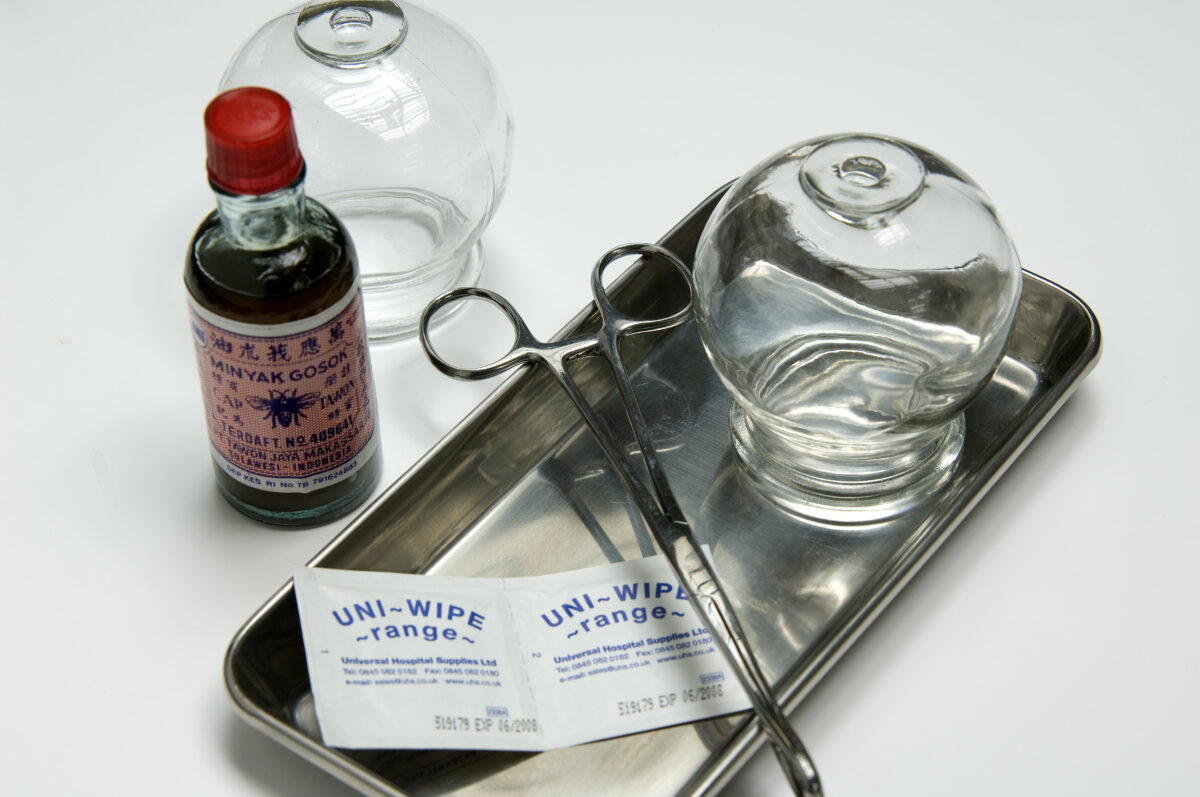The indoor photograph showcases a collection of medical equipment meticulously arranged on a white table. Centered in the composition is a silver metal tray with a slightly elevated lip, containing various items essential for medical procedures. In the tray lies a pair of stainless steel forceps and a small metal cup or bowl turned upside down. Below these are two unopened white packets labeled "Uniwipe Range Universal Hospital Supplies Ltd," with an expiration date in June 2008. Adjacent to the tray on the left, another identical metal cup is visible, and in front of it stands a small glass bottle filled with a dark liquid. This bottle features a red lid and a predominantly pink label with dark blue text that reads "Minyak Gosan" and includes an illustration of an insect, flanked by the words "Cap Tuan." The composition radiates clinical precision, with a pure white backdrop enhancing the sterile and organized ambiance.